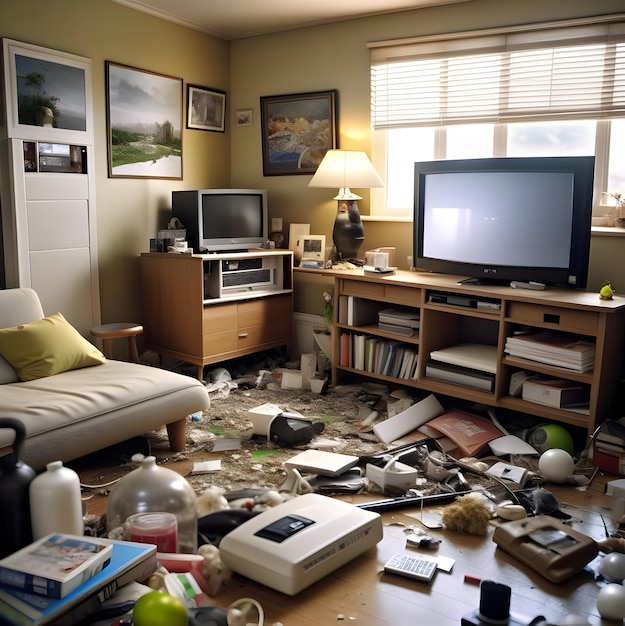This photo captures the inside of a messy, cluttered room with a wooden, brown floor strewn with various items, including papers, books, electronics, balls, and broken objects. To the left side, near a yellow-painted wall, stands a white sofa adorned with a yellow pillow. Opposite this, on the right side wall, there is a large window with white blinds that allow light to pour into the room. Below this window, a TV is placed on a light-colored dresser. Further right, another bookcase supports a large TV, placing emphasis on the multiple electronic devices scattered around. Overall, the pale yellow walls and the small visible section of the beige ceiling at the top enhance the room's slightly disorganized yet well-lit appearance.